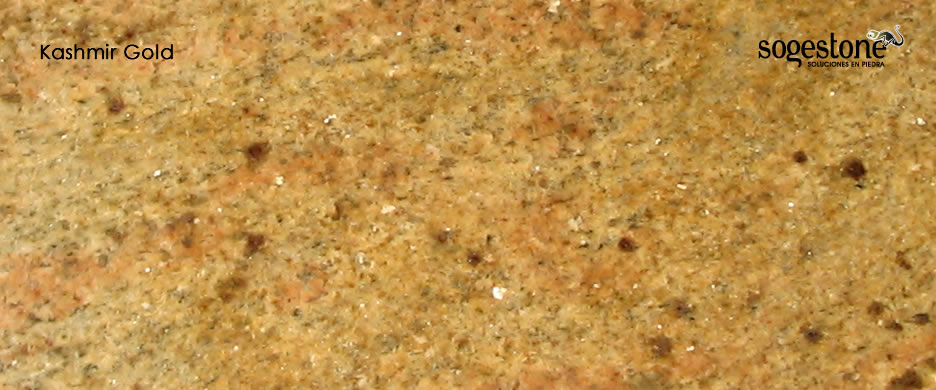The image displays a close-up of a stone or granite countertop, primarily golden in color with intricate textures. The countertop features an array of shiny white and brown specks, interspersed with areas of slightly darker or lighter stone in brownish and yellowish hues, creating a vibrant and detailed surface. On the top left-hand side of the image, in clear black text, is the brand name "Kashmir Gold." The top right-hand side features the word "Sojastone" in lowercase, stylistic black text, with the smaller words "Soluciones" and "Piedra" directly beneath the latter portion of the word "Sojastone." Notably, a small cartoon-style chameleon, colored black and light green, clings to the right side of the letter "E" in "Sojastone," adding a playful element to the otherwise elegant design. The natural light enhances the clarity and brilliance of the countertop, making its golden beige and brown shades vividly stand out.